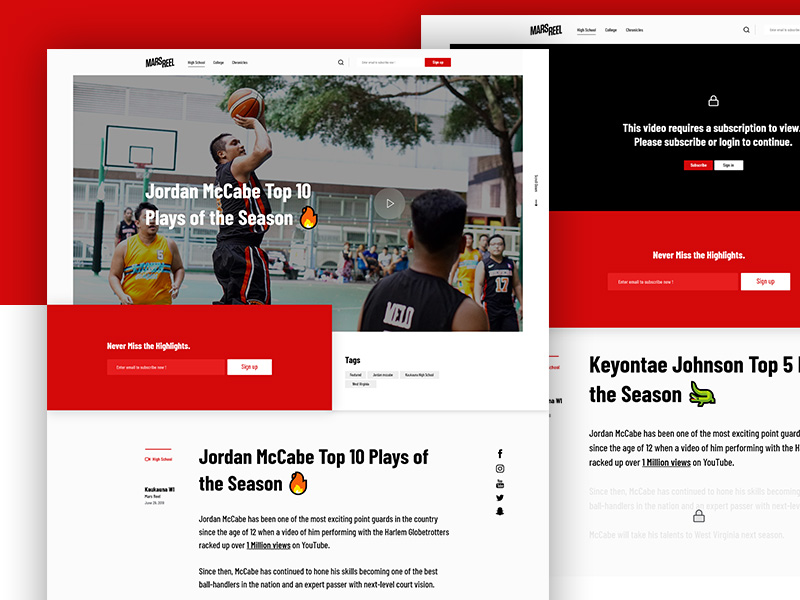The image is a collage showcasing content from the website "Mars Reel." The background features a red and white color scheme. In the foreground, a page is prominently displayed on the left, highlighting an article titled, "Jordan McCabe: Top Ten Plays of the Season."

The article features an image of Jordan McCabe, who is depicted mid-jump shot in a casual setting. He appears to be playing pickup basketball in a Southeast Asian country. Despite the informal setting, the caption notes that he is one of the most exciting point guards in the country, currently in Siege of Twelve. An embedded video from his performance with the Globetrotters has garnered over a million views on YouTube. McCabe is clad in a black jersey, while his opponent wears a yellow one, suggesting some level of organized adult league play.

On the right side of the collage, another page focuses on "Keontae Johnson: Top Five Plays." The top of this segment contains a note that the video content requires a subscription to access, urging users to subscribe or log in.

The website "Mars Reel" appears dedicated to showcasing basketball highlights but requires an account for full access to content.